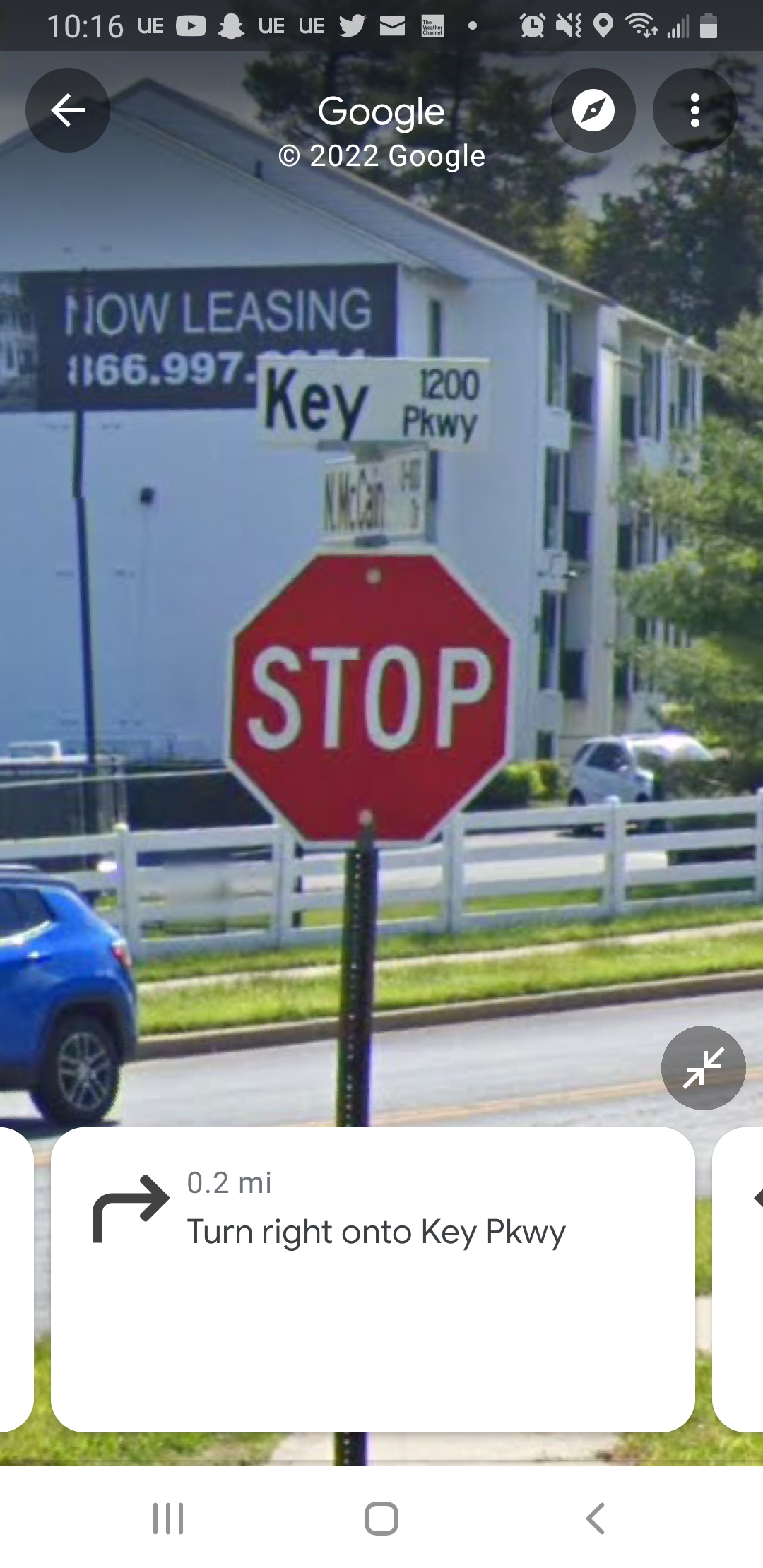In the foreground, a classic red stop sign with white lettering stands prominently, its octagonal shape clear and unmistakable. Just above the stop sign, an additional sign reads "Key Parkway" and "1200 McCann" in neat print. Beneath the stop sign, another small white sign provides directional guidance, instructing drivers to "Turn right onto Key Parkway" in 0.2 miles, complete with a right-pointing arrow for clarity. 

In the background, a cluster of modern apartment buildings is visible, surrounded by a clean, white picket fence. The apartments are accompanied by a "Now Leasing" sign, indicating vacancies. A bright blue car is seen driving down a road a short distance away from the apartments, adding a sense of movement to the scene. The sky above is clear, giving the whole setting a bright and inviting atmosphere. The overall composition suggests someone may be using a smartphone or another device to navigate the area.